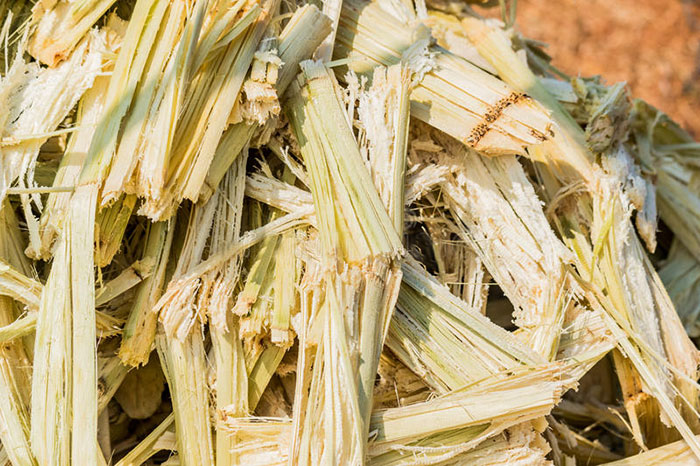The photograph, taken in bright sunlight, showcases a large pile of fibrous plant stalks, possibly sugarcane or similar cane-like plants, that have been broken up and stacked together. The stalks, mostly light green but also interspersed with whitish, straw-like pieces, display an array of textures, particularly fibrous interiors exposed due to the breakages. Some pieces are long and cylindrical, while others are shorter and more fragmented. The image is tightly populated with these stalks, filling the frame with their intertwined forms. In the background, a small triangular section of red dirt is visible, slightly out of focus, contrasting with the primarily green and white subject matter. The photograph is a detailed representation, capturing both the bright outdoor lighting and the intricate details of the plant material.